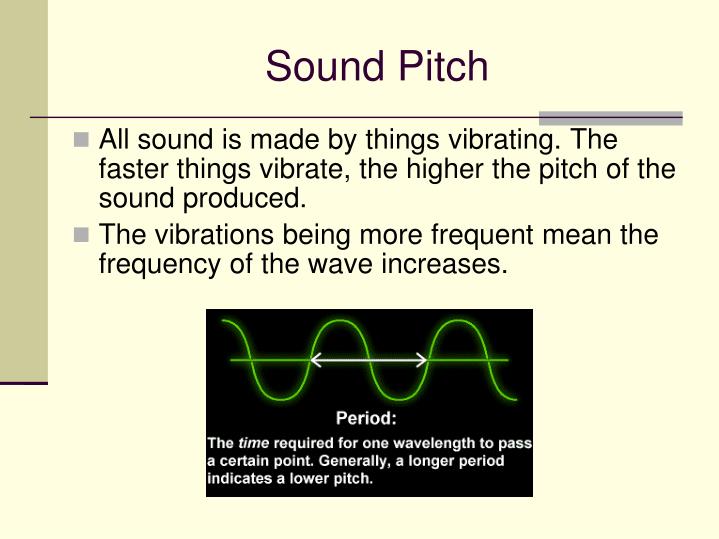This PowerPoint slide titled "Sound Pitch" features a detailed explanation of sound pitch, set against a light pink background. The title is centered at the top in black letters, underlined by a horizontal purple line. To the left, a vertical gray rectangle extends just past the midpoint of the slide. Two points are presented as gray square bullet points:

1. **All sound is made by things vibrating. The faster things vibrate, the higher the pitch of the sound produced.**
2. **The vibrations being more frequent mean the frequency of the wave increases.**

Beneath these points, a black rectangle centered on the slide displays a visual representation of sound waves as a green line oscillating in a sine pattern. This image is labeled "Period:" in white, with an explanation below: "The time required for one wavelength to pass a certain point. Generally, a longer period indicates a lower pitch." A white arrow overlays the horizontal green line, emphasizing the concept of wavelength. This detailed overview combines both textual and visual elements to explain how vibration frequency affects sound pitch.